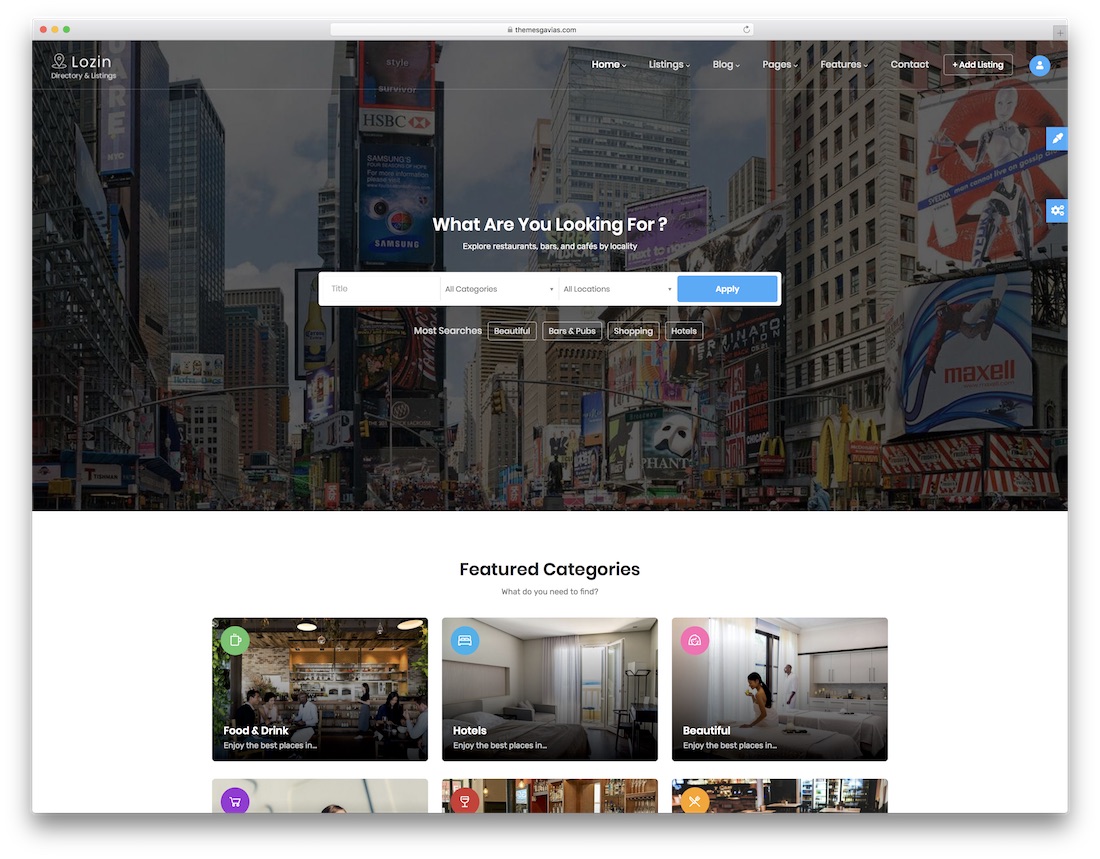Screenshot of the LOZIN Travel App Interface:

This screenshot showcases the LOZIN travel app's user interface on a computer. In the top left corner, the LOZIN logo is prominently displayed, accompanied by small text that reads "Directory" and "Listings." 

Across the top of the screen, a navigation menu features various options: 
- Home 
- Listings 
- Blog 
- Pages 
- Features 
- Contact 
- Ad Listing (highlighted with a square)
- Profile (blue and white icon for log-in)

The primary visual element of the interface is a darkened, urban backdrop, potentially depicting New York City. The scene includes high-rise buildings, multicolored lights, and advertisements for shows, creating a bustling city atmosphere. This backdrop emphasizes the search functionality in the foreground.

Central to the interface, large white text reads: "What Are You Looking For? Explore Restaurants, Bars, and Cafes by Locality." Below this search prompt is a search bar for users to input their location. Underneath the search bar, a suggestion text states, "most searches are beautiful," and keyword options like "Bars and pubs," "Shopping," and "Hotels" are also provided.

The lower half of the screen transitions to a white section featuring categorized tiles. A heading reads "Featured Categories," and the visible tiles include:
- Food and Drink
- Hotels
- "Beautiful" (illustrated with an image suggestive of a spa)

Three additional tiles are present but not fully visible in the screenshot. The well-structured layout and aesthetically appealing design make navigation and functionality of the LOZIN travel app user-friendly and engaging.